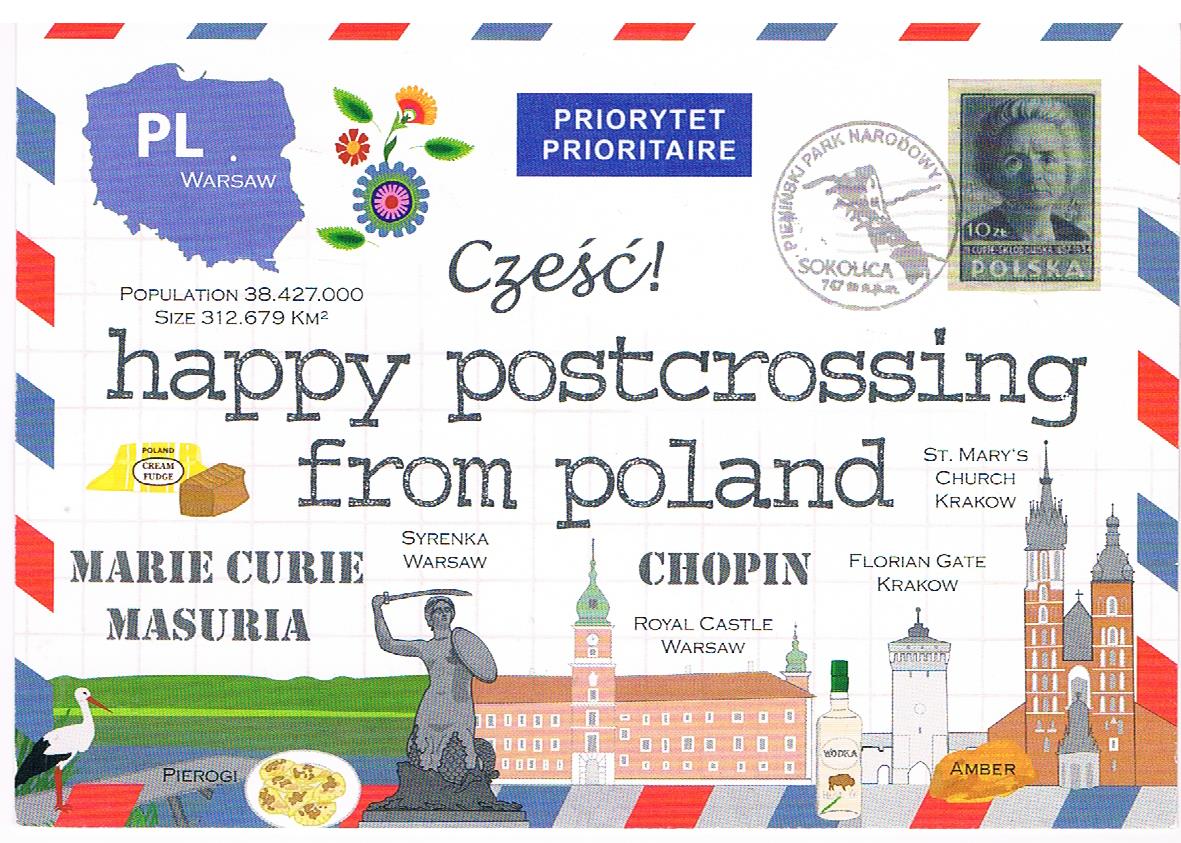This image resembles an old postcard likely from the 1970s or 1980s, prominently featuring Polish culture and landmarks. The postcard's border is reminiscent of a barbershop pole with twisting white, red, and blue stripes. Central to the design, in large, lowercase text, is the greeting, "happy post-crossing from Poland."

Surrounding this central message are various cartoonish illustrations and factual snippets detailing significant aspects of Poland. Starting from the top left and moving clockwise, the postcard includes:

- A blue outline of Poland marked with "PL" and labeled with the country’s population of 38,427,000 and its size of 312.679 square kilometers.
- A depiction of Warsaw alongside a map of Poland.
- The word "CZEŚĆ!" (Hello) with an exclamation point, "Prioritate," a postmark, and a "Polska" stamp.
- An image of St. Mary's Church and Florian Gate, both located in Krakow.
- Visual representations and mentions of Polish elements such as amber, vodka, the Royal Castle in Warsaw, and a statue of Schränka, Warsaw featuring a woman with a sword and shield.
- Labels for traditional Polish items: pierogi, cream fudge, and a nod to Marie Curie.
- Finally, a mention of Masuria, a region in Poland known for its lakes.

The combination of these elements vividly conveys the rich cultural and historical heritage of Poland.